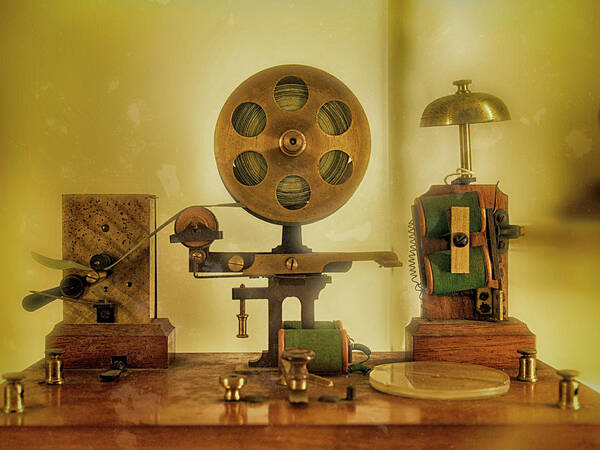The image depicts a collection of intricate vintage equipment displayed on a shiny cherry-colored wooden table, set against a bright yellow background. On the left, there's a brown wooden box featuring a rectangular component with black knobs and a piece of tape running to the center. This middle section consists of a metallic dark brown base adorned with a gold strip, topped by a circular wheel with tape, possibly indicating a film device. Adjacent to this, on the right side, stands a gold bell next to another wooden box with a green element trimmed in brown. Scattered across the table are numerous brass and gold knobs, including two on both the left and right sides, a central circular gold element with a lever, suggesting these might be parts of the equipment or decorative accents. The overall setup evokes a sense of antique technological complexity amidst a richly colored backdrop.